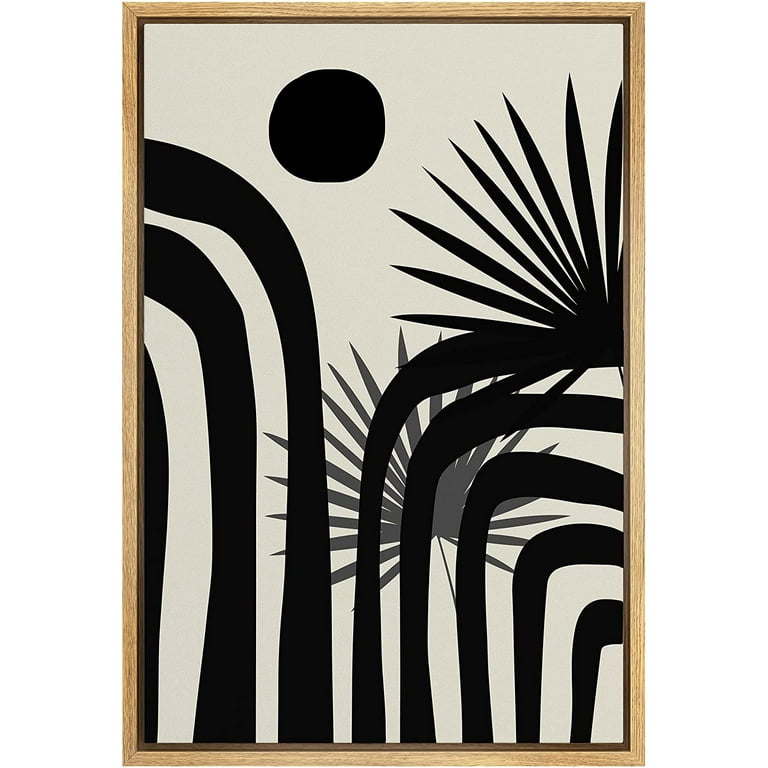The painting, encased in a simple, light-toned wooden frame, presents a striking abstract composition. The background features a blend of light gray, cream, and off-white hues. At the top left, there is a slightly deformed black circle, reminiscent of a sun or moon. Stark black curves streak from the left side and extend down to the bottom, mirroring a similar pattern of dark curves emanating from the right. Near the center, a black palm frond stands out, while a gray version of the same palm frond subtly merges into the background. The piece, an elongated vertical rectangle, exudes a monochromatic zebra-like aesthetic, with the black and gray imagery contrasting vividly against the light backdrop.